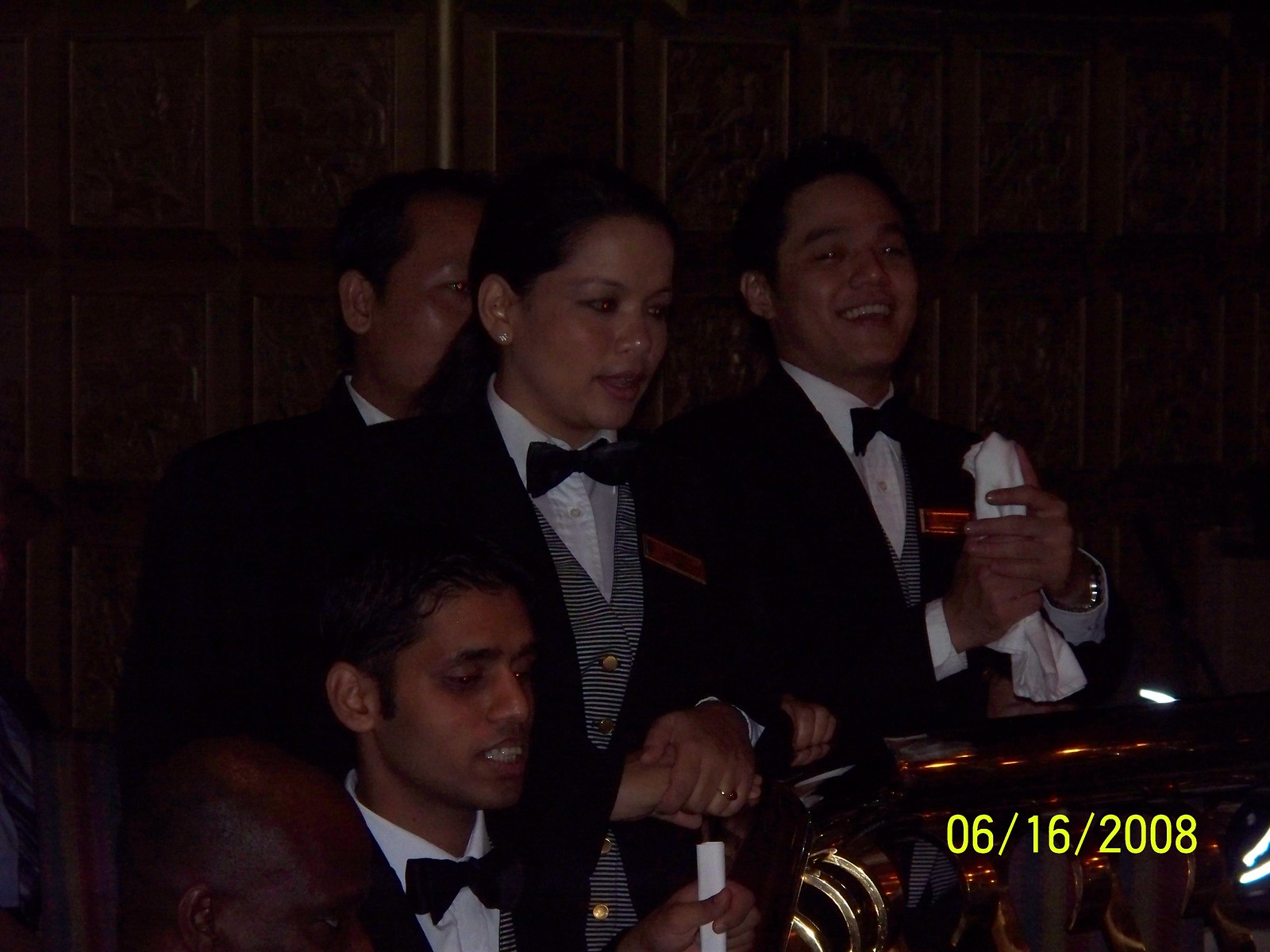In the image dated June 16, 2008, four individuals dressed in formal attire stand in what appears to be a ceremonial or solemn setting, possibly a church or similar location, characterized by a large wooden door in the background. Each person is wearing a black tuxedo with a gray and white striped vest adorned with gold buttons and a bow tie, along with a nameplate or badge on their jackets. 

To the right, a boy is smiling while holding a white napkin pointed upward. To his right stands a woman with black hair tied back, ear studs, and her hands clasped and resting on a dark brown or dark gold railing behind them. Below her, kneeling and appearing solemn, is a man who holds an unlit white candle, possibly indicating a religious ceremony. There is also a partial view of another individual, whose head alone is visible and who appears to be a Black man, suggesting there are more people present in the setting. The overall atmosphere suggests that the image captures a special occasion or celebration with a dignified and possibly religious tone.